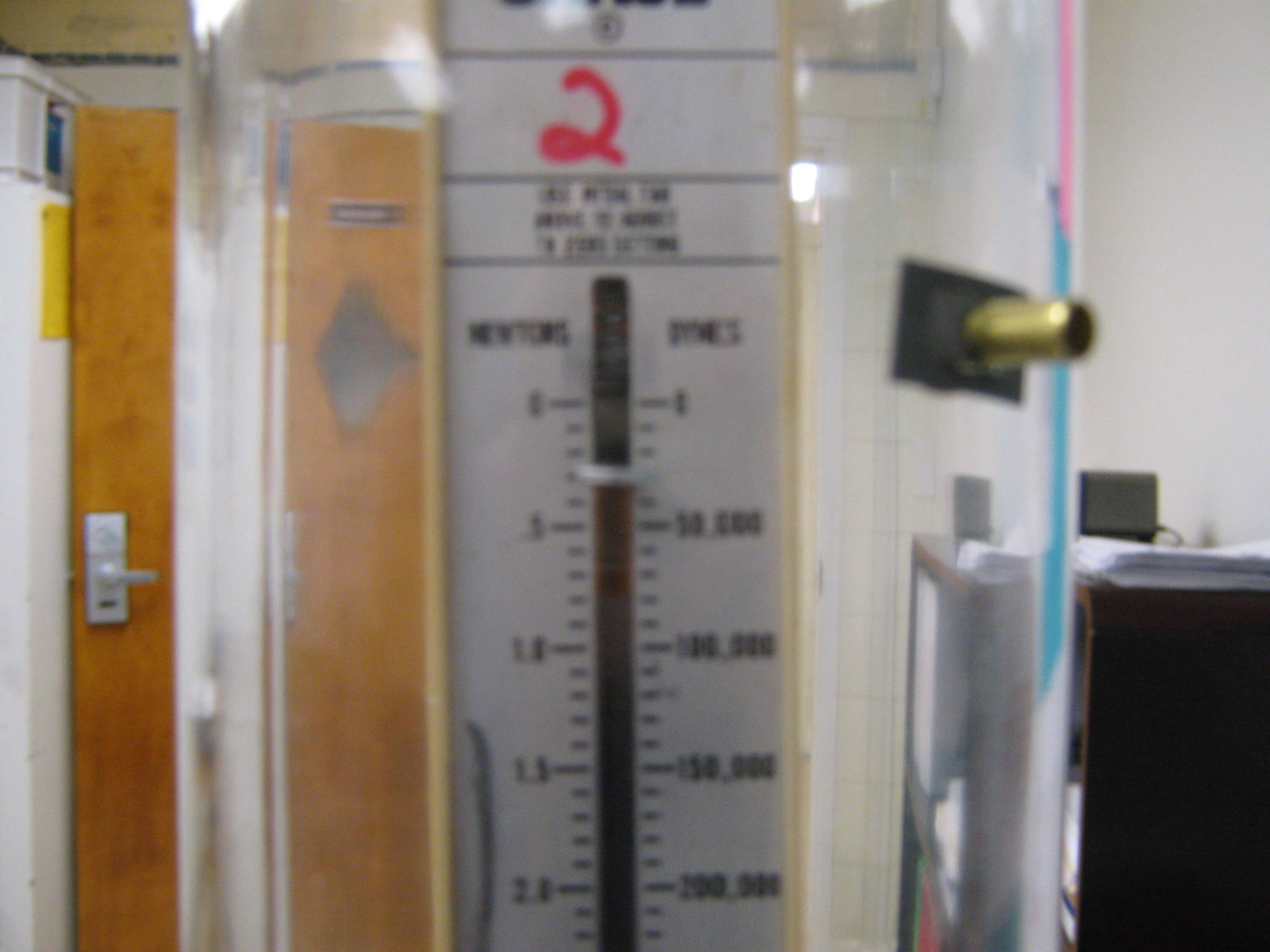The room features very light gray walls and two brown wooden doors. Positioned beside one door is a white hot water heater, adorned with a prominent yellow sign and topped with a white box. An oversized white thermometer with black markings and a red number two at the top hangs nearby, enclosed within two pieces of glass. To the right, part of a sink or cabinet is visible, with a small black box placed atop it, connected by a wire. A piece of glass on the side of the thermometer is framed by a black wooden strip, from which a small gold pipe protrudes.